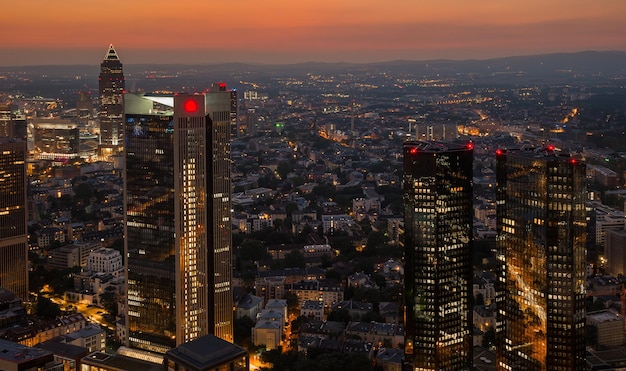The photograph captures a stunning aerial view of a city's skyline just after sunset, with the dim pinkish-red sky framing the scene. In the foreground, five prominent high-rise buildings stand out, each around 30 to 40 stories tall. One building on the very left is particularly noticeable, followed by another slightly to its right; two more dominate the right-hand side of the image. Another substantial building is slightly off to the left, set against a backdrop of smaller, lower structures. The tallest buildings reflect a golden tint, possibly from the setting sun, and are adorned with red lights on their tops, adding a dramatic flair. Numerous twinkling lights emanate from the windows of both the tall and smaller buildings, enhancing the city’s urban charm. The overall lighting is carefully balanced, giving an amber hue to the photograph, which enhances its high-quality appearance. The distant horizon reveals a faint outline of mountains, adding depth to the already picturesque cityscape.